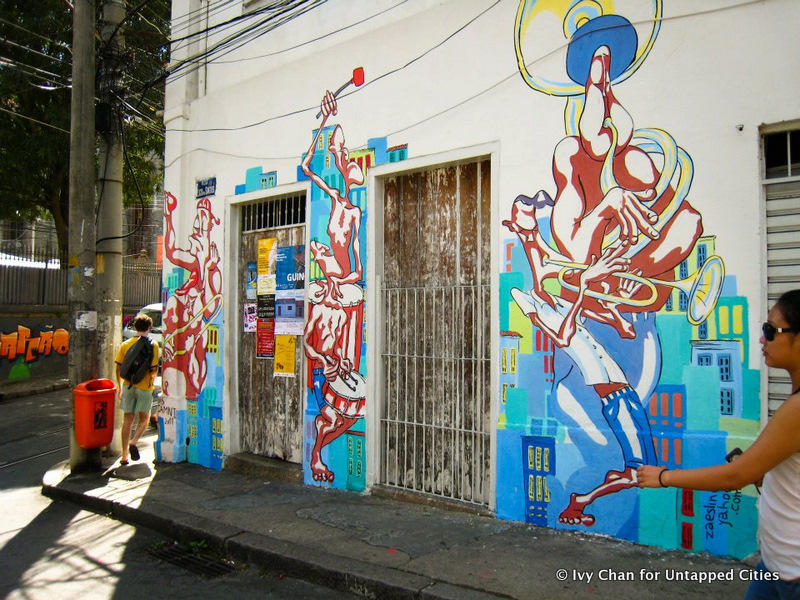This photograph captures an urban scene featuring the side of a white stucco building, reminiscent of architectural styles found in Mexico, Central America, or South Texas. Distinctive for its vibrant, graffiti-style murals, the artwork includes disproportionally drawn figures playing musical instruments—trumpets, drums, and another indeterminate instrument. The murals evoke a nostalgic 1970s "keep on truckin'" aesthetic. The windows and door of the building are secured with iron grates, and the door itself is plastered with numerous, unreadable advertisements. The image also captures two pedestrians: a woman in a sleeveless shirt and sunglasses walking on the far right, and a boy with a backpack rounding the corner on the far left. A red trash can is attached to a pole on the left side, while an electric concrete post with an orange plastic container at its base stands prominently near the center. The surrounding cityscape features additional graffiti on a nearby wall, characterized by colorful words in orange and green. The image is labeled in the bottom right corner as "Ivy Chan for Untapped Cities."